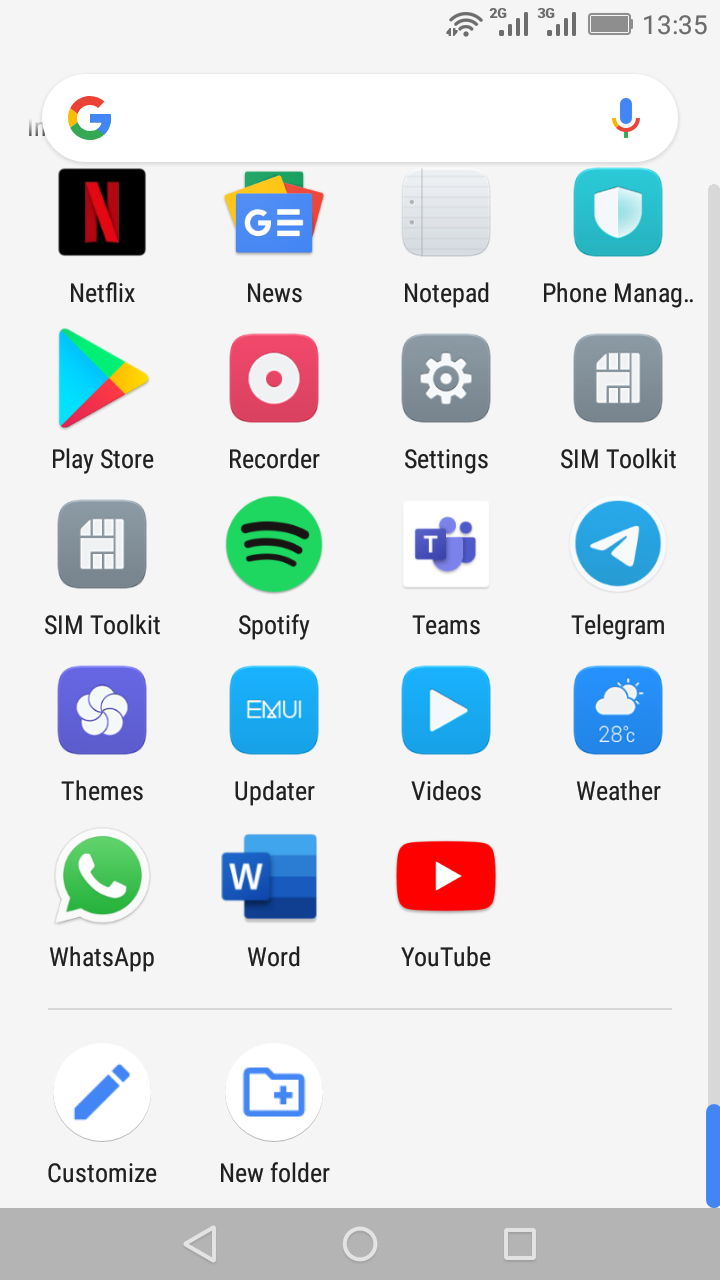The image shows a detailed screenshot of a smartphone interface, set against a gray background. At the top of the screen, the status bar displays various indicators: a 2G network connection is active with a strong signal, 3G is also available at four bars of strength, the battery is fully charged at 100%, and the clock shows military time as 13:35 (1:35 PM). Below the status bar, a Google search bar is open, identifiable by the prominent Google "G" logo.

The main portion of the screen features five rows of app icons with their names. This appears to be an imaginary mock-up rather than a depiction of a real phone. The detailed breakdown of the app icons by row is as follows:

**Top Row (from left to right):**
1. Netflix
2. Google News
3. Notepad
4. Phone Management

**Second Row:**
1. Google Play Store
2. Recorder
3. Settings
4. SIM Toolkit (duplicated twice)

**Third Row:**
1. Spotify
2. Microsoft Teams
3. Telegram
4. Themes

**Fourth Row:**
1. Updater
2. Video
3. Weather

**Fifth Row:**
1. WhatsApp
2. Microsoft Word
3. YouTube

The clean, organized presentation of app icons against the monochromatic background gives the interface a polished and uniform appearance.